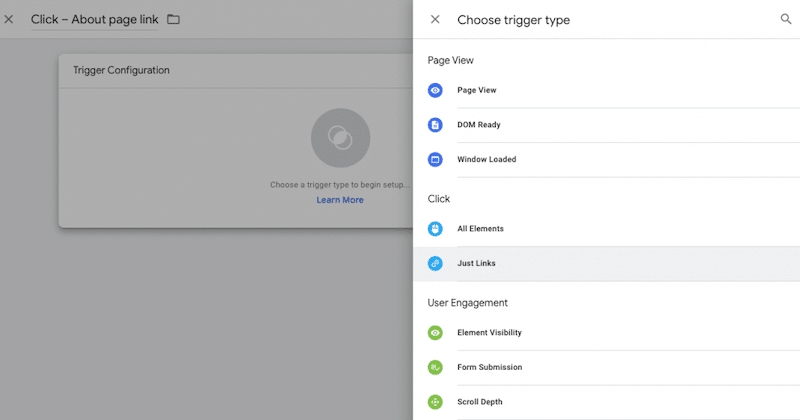The image is a detailed screenshot of the backend interface of a website or blog editing platform. The primary background is minimalistic and white, giving it a clean and uncluttered appearance. Central to the image is the main workspace, currently blank with a placeholder prompt indicating where content can be added later.

On the right side of the interface, a dropdown side menu is visible, displaying a list of functionalities including "Page View," "DOM Ready," and "Window Loaded." Each option is accompanied by a colored icon: dark blue for page views, light blue for DOM ready, and green for window loaded. These icons include simple symbols, such as an eye for page views, a folder for DOM ready, and a document icon.

Further down the menu, there are additional options under the "User Engagement" section, which lists items like "Element Visibility," "Form Submission," and "Scroll Depth," indicating tools for tracking user interaction with the content.

Overall, the layout is intuitive and focused on providing essential tools for website or blog creation without overwhelming with excessive color or intricate details.